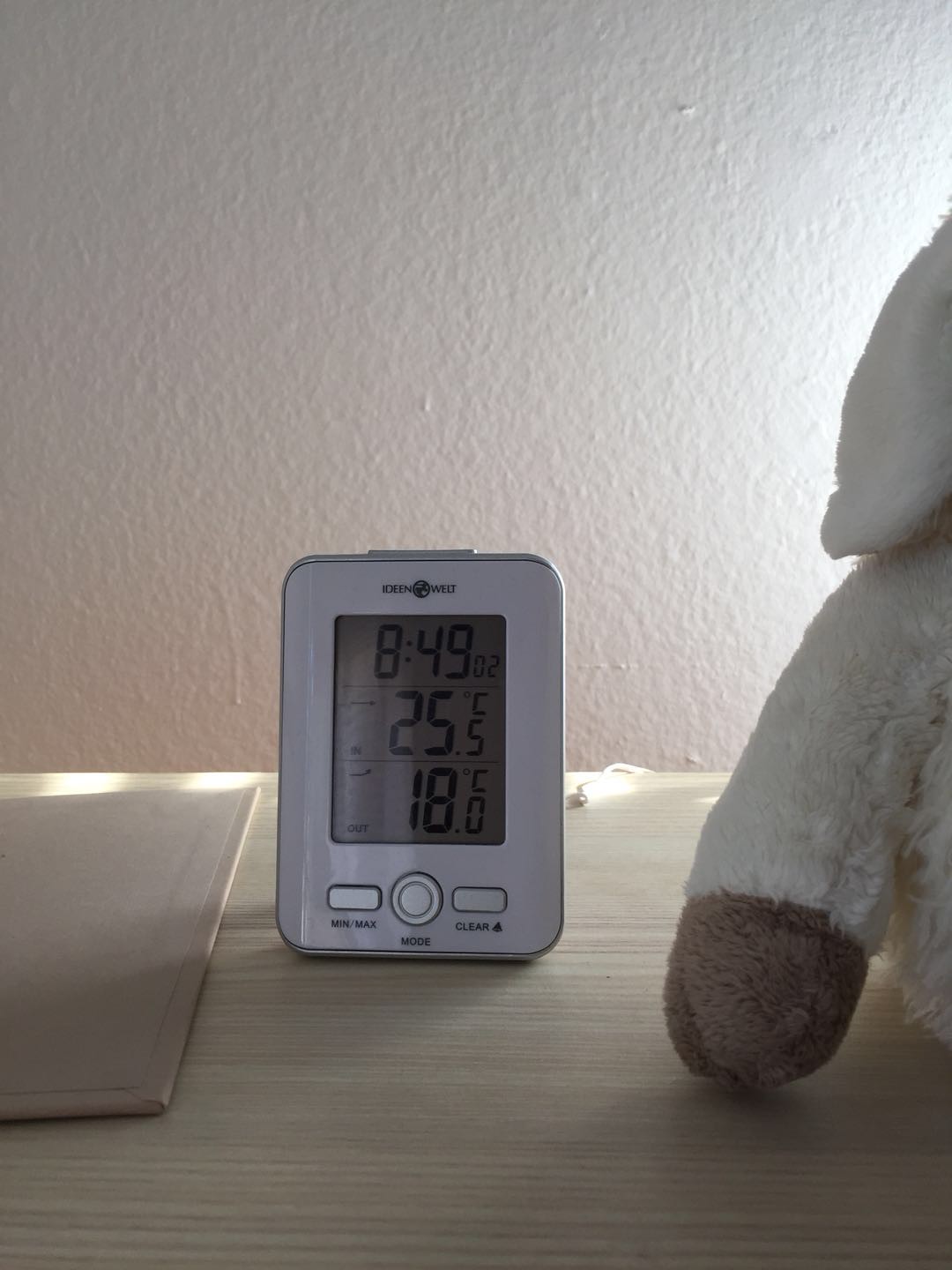The image features a vertically aligned, portrait-mode photograph showcasing a digital monitor on a light wooden tabletop, the grains of which run horizontally across the frame. The backdrop is a plain white wall, illuminated by a light source emanating from the right side of the image. A partial view of a stuffed animal, characterized by its white fur, brown hand, and visible ears, appears along the right edge of the photo.

At the center of the scene stands a digital monitor with an LED display. The display features a gray background, with bold black numerals reading "849" followed by "02 seconds". Below these numbers, the display indicates the temperature readings: "25 Celsius" followed by "18 Celsius". The monitor itself is white and is equipped with several buttons labeled "minimum", "maximum", "mode", and "clear".

Adjacent to the monitor lies a downturned picture frame, clad in a beige hue, adding an additional element of interest to the composition.